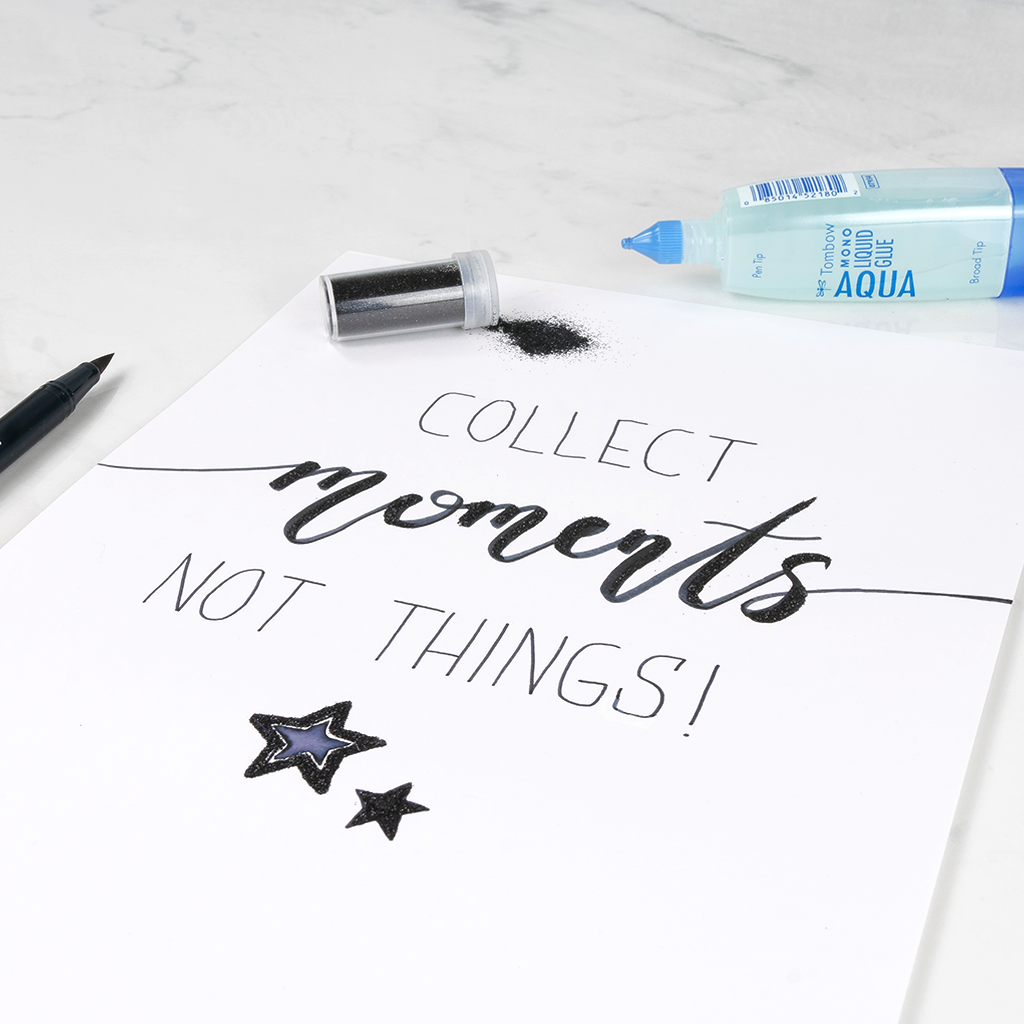The photograph showcases a white marble countertop on which a handwritten sign rests. The sign reads, "collect moments, not things!" in varying fonts: "collect" is in a lighter, standard print, "moments" is emphasized in bold cursive, and "not things!" is in block letters with an exclamation point. Glitter has been purposefully scattered across the top of the sign, notably above the word "collect," creating a sparkly effect. Below "not things!" there are two stars: the left one has a purple interior with a black outline, and the right one is entirely black.

To the left of the sign, there is an uncapped black pen, and near the top, a tipped-over black glitter bottle has caused a spill. On the right side, a clear, Aqua Mono liquid glue bottle by Tombow lies on its side, identifiable by the label with a barcode. This scene, with its various art supplies and detailed lettering, gives the impression of a creative craft project in progress.